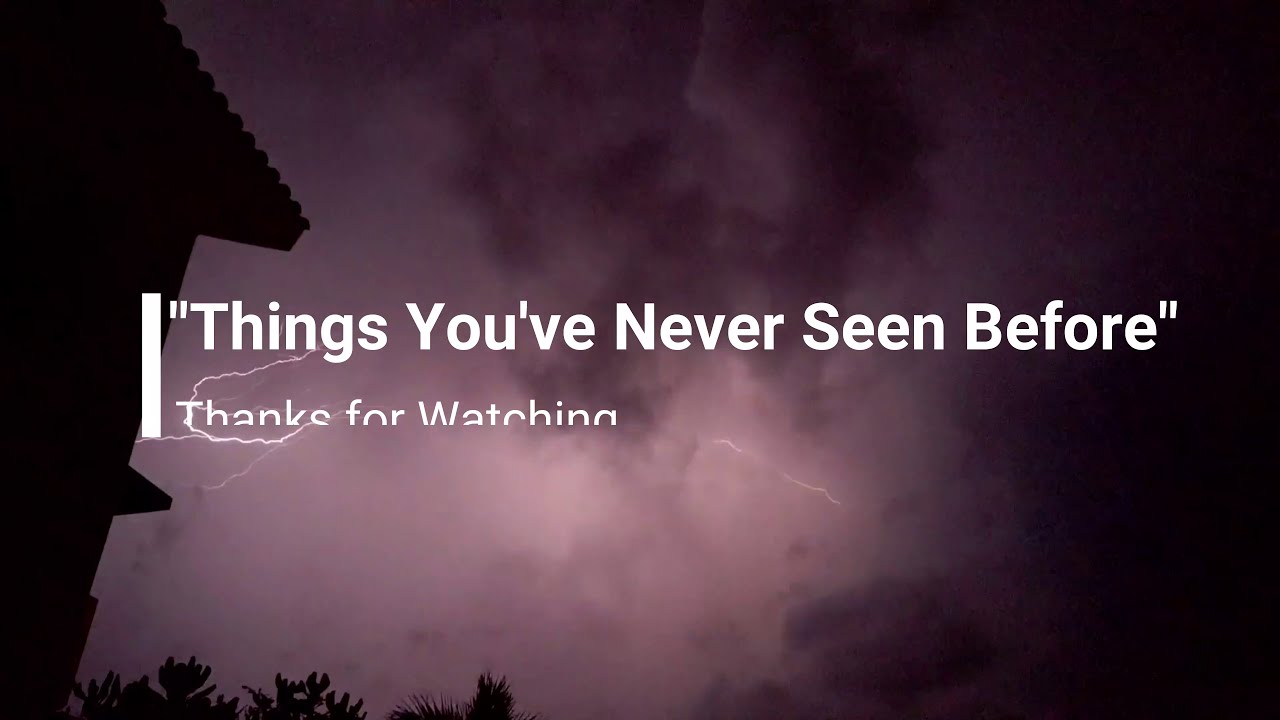In the center of this image, bold white text reads "Things you've never seen before," with thinner white text below it stating "Thanks for watching." Both texts are aligned by a white line that extends vertically from the top to the bottom of the text block. The backdrop features an ominous storm with dark, roiling clouds and a vivid lightning strike emanating from the center and extending to the right, slightly branching to the left. Subtle hues of deep purples and grays color the sky, enhancing the dramatic scene. In the bottom left corner, the silhouetted outline of a building with visible roof shingles is partially shrouded by smokey, storm-induced haze, and flanked by bushes or trees, further contributing to the tumultuous atmosphere.